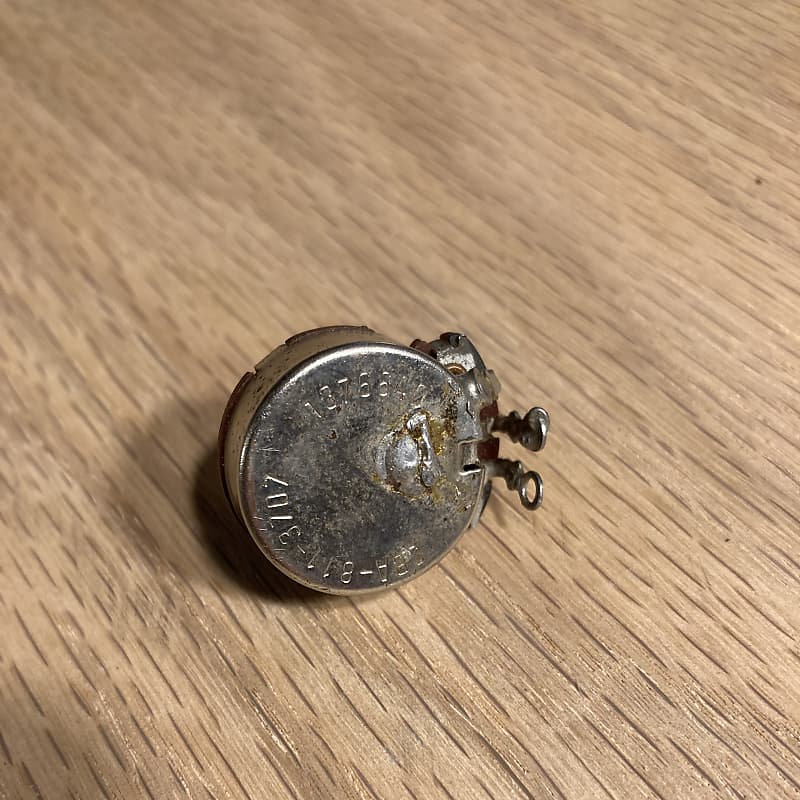The photograph features a small, circular, silver electrical device, likely a potentiometer or variable resistor, situated on a brown, striped tabletop. The table exhibits narrow black and dark brown streaks running in various directions. The silver object, which shows signs of wear and some rust or brown stains, prominently displays some engraved letters and numbers, although only "811-3707" and "18766" are discernible. The device has a width estimated between a quarter to half an inch and includes two metal attachments on the right side that appear to facilitate electrical connections. While the image is zoomed in, giving a detailed view of the object, the lack of other items for scale makes it challenging to accurately determine its precise size. The object is clearly the focal point, with its circular shape and engraved details drawing immediate attention.